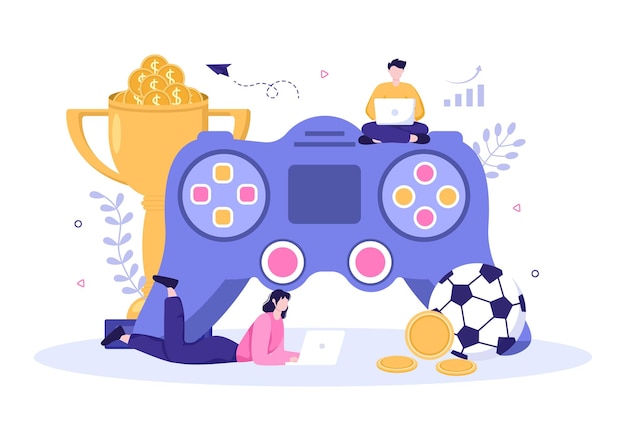This detailed, computer-generated image features a large, PlayStation-like game controller at its center, colored in a striking blue with distinctive pink and yellow buttons—square ones on the left and round ones on the right. The analog sticks are also pink. Sitting atop the oversized controller is a man dressed in a yellow shirt and purple pants, engaged with his laptop. Below him, on the floor, a woman in a pink long-sleeved shirt and purple pants similarly concentrates on her laptop, suggesting a collaborative or recreational digital activity. 

To the bottom right of the controller lies a classic black-and-white soccer ball with three gold coins positioned in front of it. Behind the controller, slightly to the left, stands a gleaming trophy brimming with gold coins. The background is minimalistic with various whimsical elements like looping dotted lines and a small paper airplane on the left side, adding to the playful and eclectic feel of this animated scene.